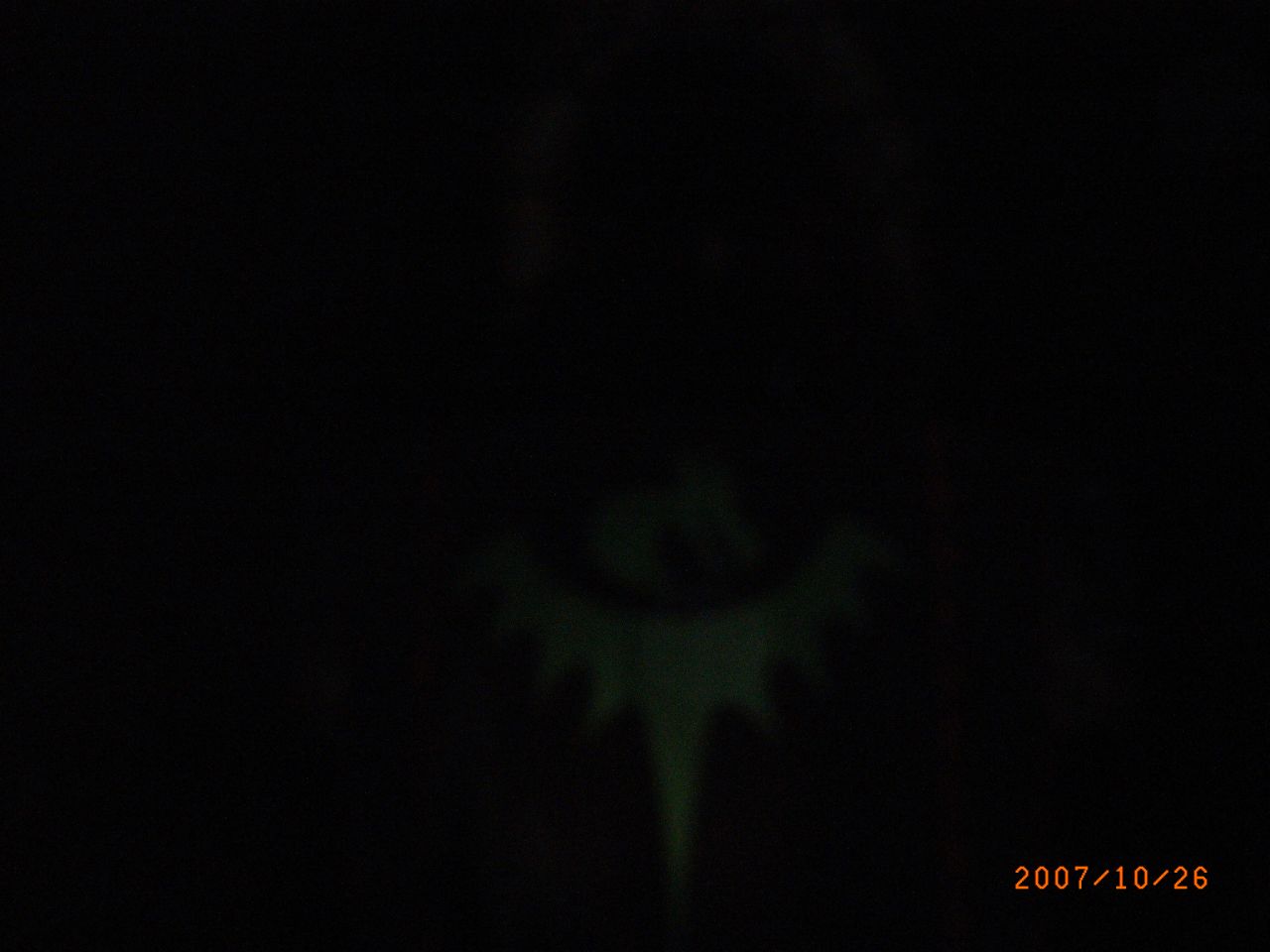This extremely grainy, horizontally-oriented color snapshot photograph initially appears entirely black. However, hidden within the darkness is an obscure object beneath the center midpoint, resembling an inverted crown. This crown-like shape, with its tall, steeple-like point, angles toward the bottom right of the image and displays a faint dark green tint. Atop the base of this inverted crown rests a curved object. The photograph, taken on October 26, 2007, as indicated by the orange date stamp in the bottom right corner, maintains a predominantly jet-black backdrop, creating a mysterious and ethereal scene.